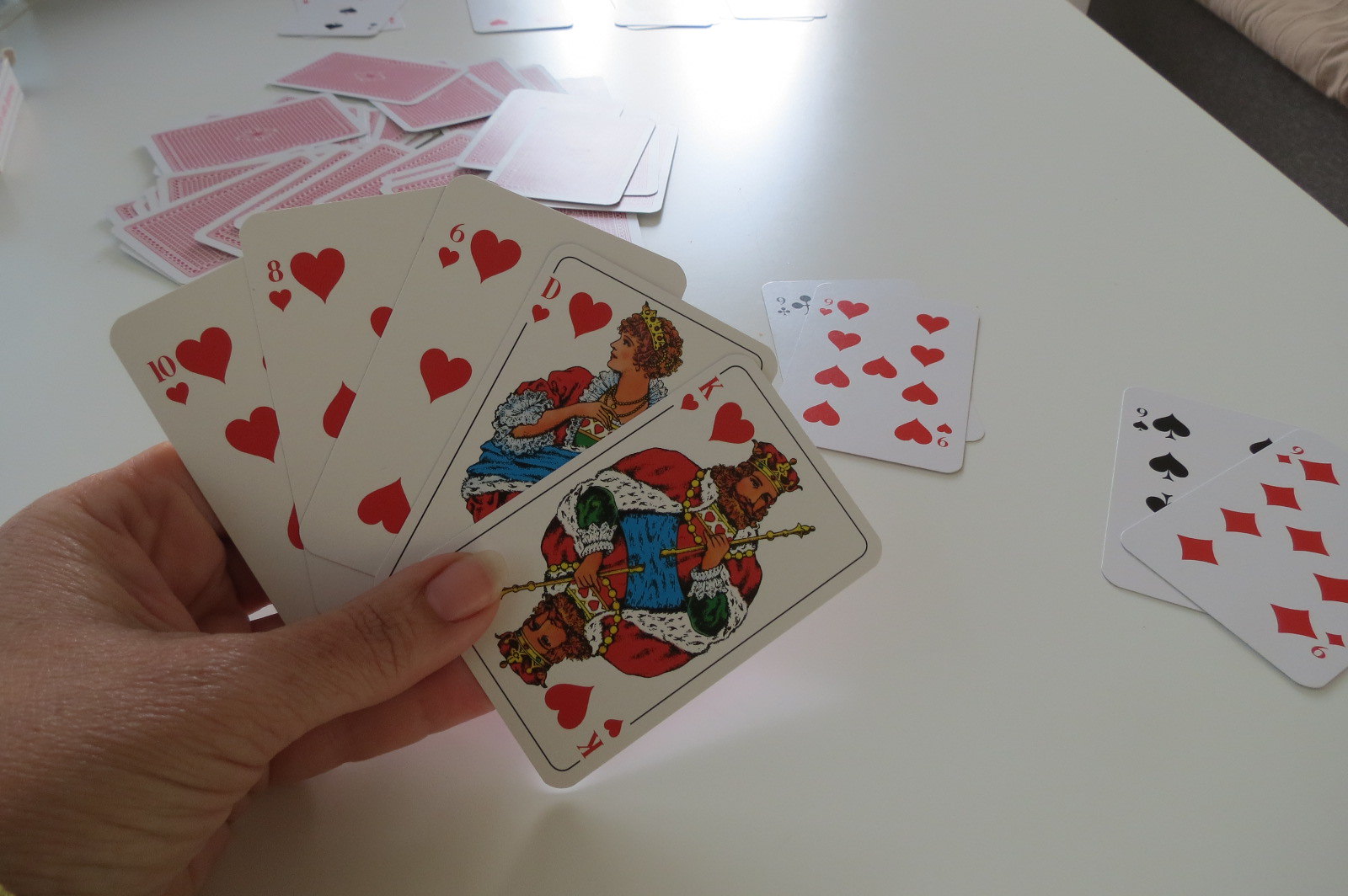The image depicts a large white tabletop scattered with playing cards. At the center of the table, a collection of cards lies face down, extending towards the far end of the tabletop. In the bottom right corner, four prominent stacks are visible. The first stack features a six of clubs topped by a six of hearts. Adjacent to it, the second stack shows a nine of spades with a nine of diamonds on top.

Additionally, a close-up reveals a person's hand holding five cards arranged like a typical poker fan. The cards are a ten of hearts, eight of hearts, six of hearts, and a king of hearts. The scene vividly captures an ongoing card game, detailing the layout and specific cards in play.